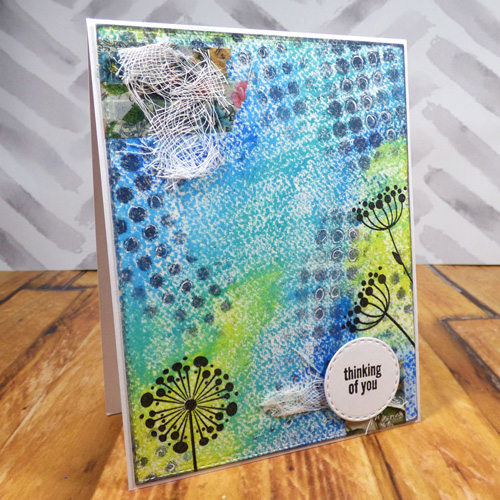This image showcases a meticulously handcrafted "Thinking of You" greeting card. The card is propped up on a rustic, brown wooden table against a backdrop featuring diagonal gray and white stripes. The card has a square shape and an intricate design. It predominantly features shades of blue, teal, and green, with accents of yellow. The background of the card exhibits a watercolor effect with dandelion seed illustrations, some appearing white and others yellow, resembling the parachutes that carry dandelion seeds.

Adding to the texture and design, there are elements that look like white lace or linen fabric, particularly noticeable in the upper left corner and near the bottom beside a small circular emblem. This emblem is a white circle with a likely leather or similar material border, prominently displaying the phrase "Thinking of You." The card appears to be partially open, suggesting that it can be personalized with a handwritten message inside. Adorning the card are delicate daffodil-like flowers and possibly a 4x4 bandage-like crisscross pattern, adding to its unique, homemade aesthetic.